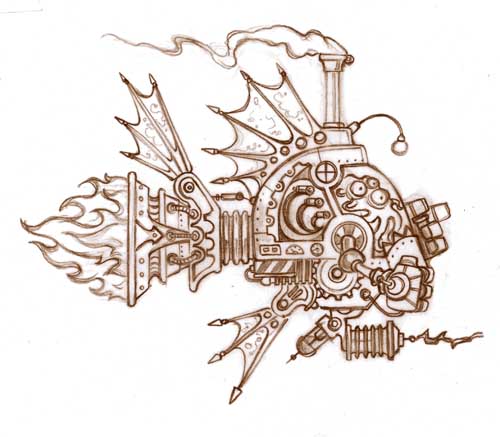This is a highly detailed sepia-tone drawing, likely done in black ink originally, depicting a steampunk-inspired, fish-shaped flying craft. The craft features prominent fins on the top, bottom, and sides, reminiscent of aquatic propulsion systems, and is adorned with an array of ornate and intricate devices. The aft section extends into a cylindrical rocket that flares into a small fish-like fin on the left, from which flames are jettisoning out, simulating a powerful exhaust system. A steam stack located on top of the craft continuously emits a stream of smoke.

The head of the fish-like vessel houses a cockpit with a glass window, revealing an alien-like octopus creature operating the controls. This creature has several tentacle-like appendages and at least three visible eyes. Dangling in front of the cockpit is an antenna-like light fixture, akin to the luminous lure of a deep-sea fish.

Additional features include three exhaust-style components at the back and two laser cannons mounted below the head—one pointing left with a curved top and another pointing straight ahead with a tapered base. The overall aesthetic, with gears, panels, cables, and attachments, evokes a fantastical steampunk machine that appears both mechanical and organic, giving the impression of a device not of this world.